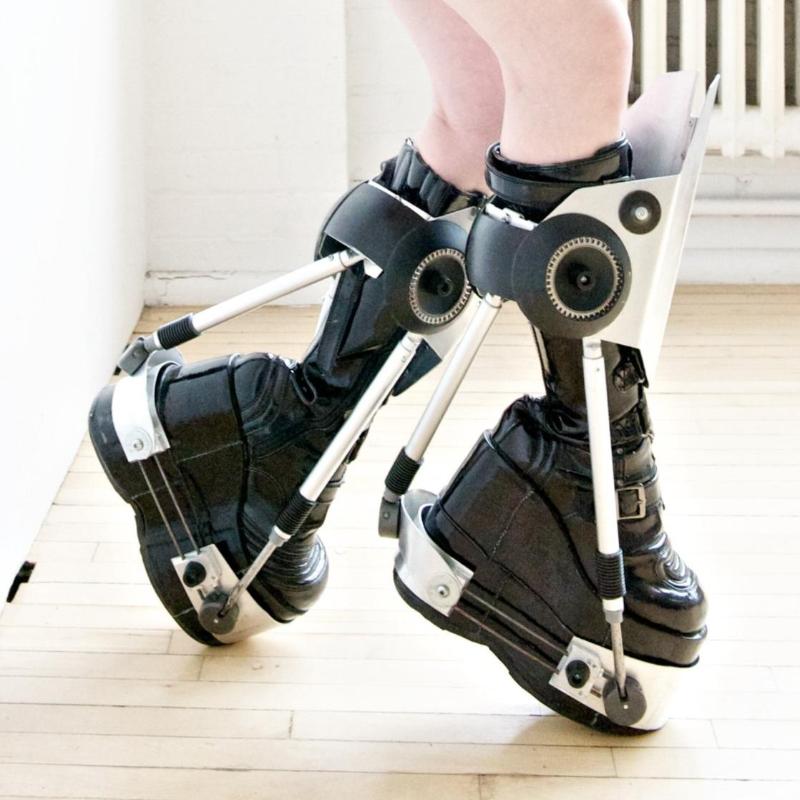The image depicts a person wearing a sophisticated orthopedic or prosthetic walking device. The device, which is primarily black and white, features knee-high boots with a mechanical, robotic aesthetic. The black shoes have buckles on the sides and substantial platforms beneath them, providing a sturdy base for walking. The device includes white knee shield guards and a metal frame built around the boots, which incorporates screws, rods, and hinges. This intricate framework connects to a gear mechanism located around the upper shin, just below the knee, likely assisting in movement and mobility. The background includes a white wall, and the floor has a tan-colored rectangular pattern, suggesting a well-lit indoor setting. The photo is taken at an angle, capturing the person from the knees down.